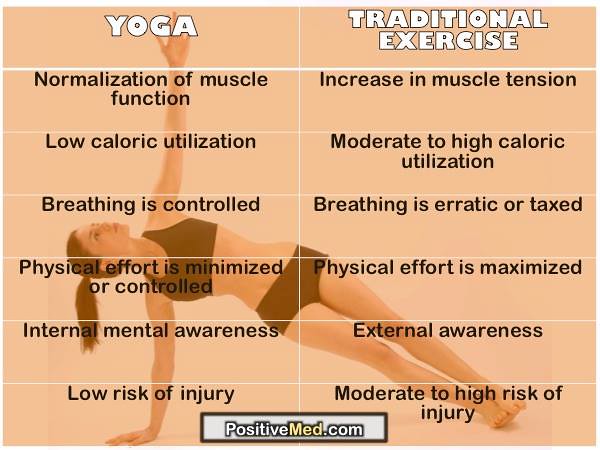This advertisement for yoga exercises features a light peach background with a fit woman performing a yoga pose. She wears a white or black top and bottom, has a dark brown ponytail, and is captured in a side plank position, balancing on one hand and feet while extending her other arm upwards. The ad compares yoga to traditional exercise through two columns of benefits and features. The left column highlights yoga's advantages, such as normalization of muscle function, low caloric utilization, controlled breathing, minimized physical effort, internal mental awareness, and low risk of injury. In contrast, the right column details traditional exercise's traits, including increased muscle tension, moderate to high caloric utilization, erratic or taxed breathing, maximized physical effort, external awareness, and moderate to high risk of injury. At the top of the image, the word "Yoga" is prominently displayed in white letters, and at the bottom middle, the website "positivemed.com" is shown against a grey background.